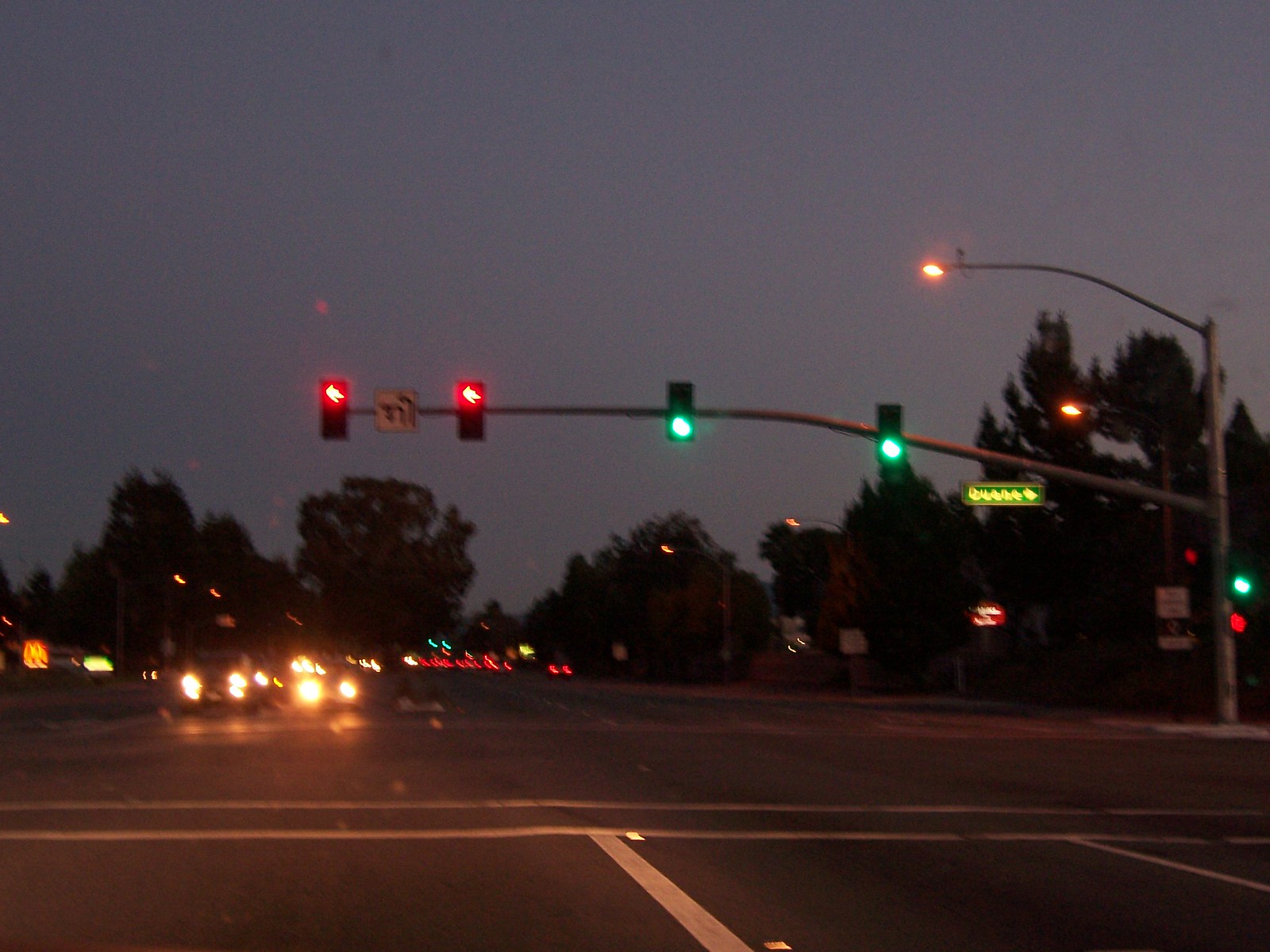This color photograph captures a bustling intersection at night. The sky is a very dark gray, suggesting it is shortly after sunset. The intersection is illuminated by several streetlights and traffic lights attached to a long gray pole. There are four main traffic lights at the intersection: two red arrows on the left indicating no left turns and two green lights to the right allowing straight passage. One additional green light is farther to the right, though its type is unclear due to blur.

Numerous cars populate both directions of the intersection. On the left-hand side, vehicles wait at the red light, with their headlights brightly shining towards the viewer. On the opposite side, past the intersection, several cars can be seen with their taillights glowing red, indicating they are either parked or moving away.

The scene also includes various street elements: a blurry street sign, a walk/don't walk pedestrian signal, and the lights of a possible strip mall in the background. Among the visible logos, a McDonald's sign is clearly identifiable on the left-hand corner. Surrounding the scene are large, dense trees lining the sidewalks, adding to the suburban or urban ambiance.

Overall, this photograph vividly depicts the nightly activity at a busy street intersection, highlighting the contrast between the bright artificial lights and the enveloping darkness of the night.